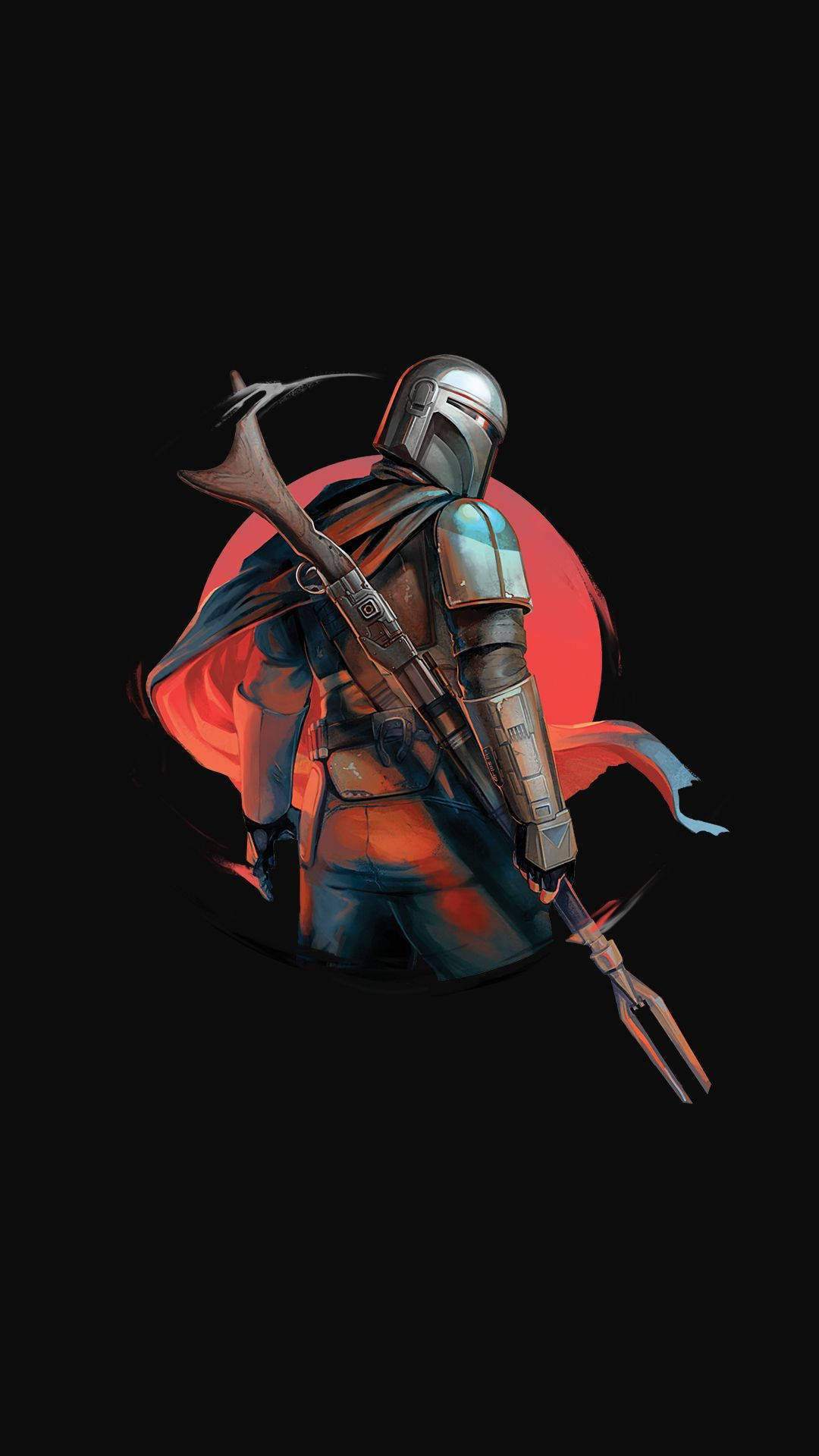Here is a cleaned-up and detailed caption for the image:

In this image, we see the Star Wars character Boba Fett captured from an over-the-shoulder perspective. Boba Fett is oriented towards the upper-right side of the frame, with his back partially facing the camera. The left arm is slightly obscured, while the right arm, prominently armored, is more visible in the foreground. His right shoulder is clad in distinctive Mandalorian armor, and both forearms are similarly armored with gauntlets that extend to cover his hands. Strapped across his back is a blaster rifle, a signature piece of his bounty hunter equipment. Boba Fett's head is turned to the right, revealing his iconic full-faced helmet made of beskar metal, its T-shaped visor facing away from the viewer. The image captures the essence of Boba Fett's imposing and enigmatic presence.